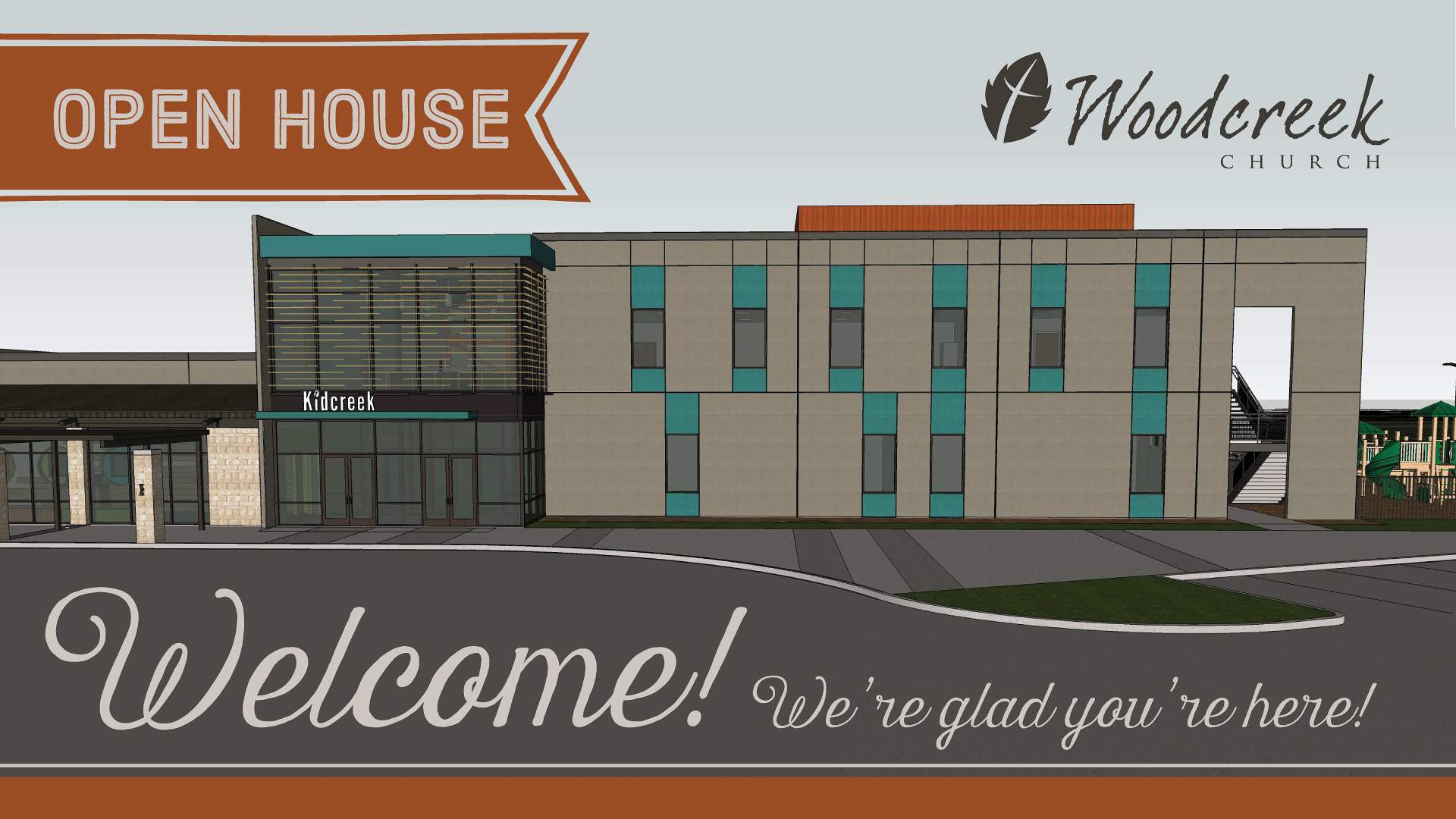The image is a digitally created advertisement for an open house at Wood Creek Church. At the top left corner, the text "Open House" is prominently displayed inside an orange ribbon. The church's logo, which features the word "Woodcreek" in a cursive script along with an illustration of a leaf and a cross, is located in the top right corner. The centerpiece of the image is a detailed architectural drawing of the church building, showcasing its modern design with extensive glass windows and an all-glass entry area. The building is depicted in shades of gray, green-turquoise, and orange. Next to the church, there is a playground area visible, adding a welcoming touch to the setting. Below the illustration, white text reads, "Welcome, we're glad you're here," with an orange border along the bottom of the image. The overall design, set against a gray background, emphasizes the invitation to the open house event and combines various warm and neutral tones to create an inviting atmosphere. The setting appears to be outdoors and gives the impression of midday light.